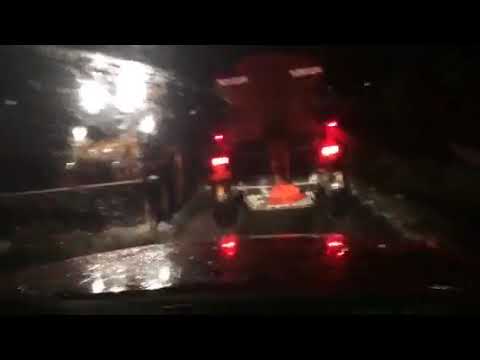The image depicts a blurry, nighttime scene focused on the rear of a large truck, possibly a semi-truck or a pickup truck, centered against a pitch-black background with black borders at the top and bottom. The truck features six red taillights—two smaller ones on the upper section and four larger ones at the bottom—along with a distinctive orange triangular sign on its rear, bordered by what seems to be a silver bumper. There is a notable glare from a white light in the upper left corner, casting a reflection on the roadway and adding to the image's overall blur. The black tires of the truck are faintly visible, and reflections of the red taillights can be seen on the ground. On the left side, there are two blurred circles of light and a white horizontal line or pole, beneath a lit area, suggesting illumination from a nearby source. The dark, almost indistinguishable surroundings underscore the difficulty in discerning more details of the scene.